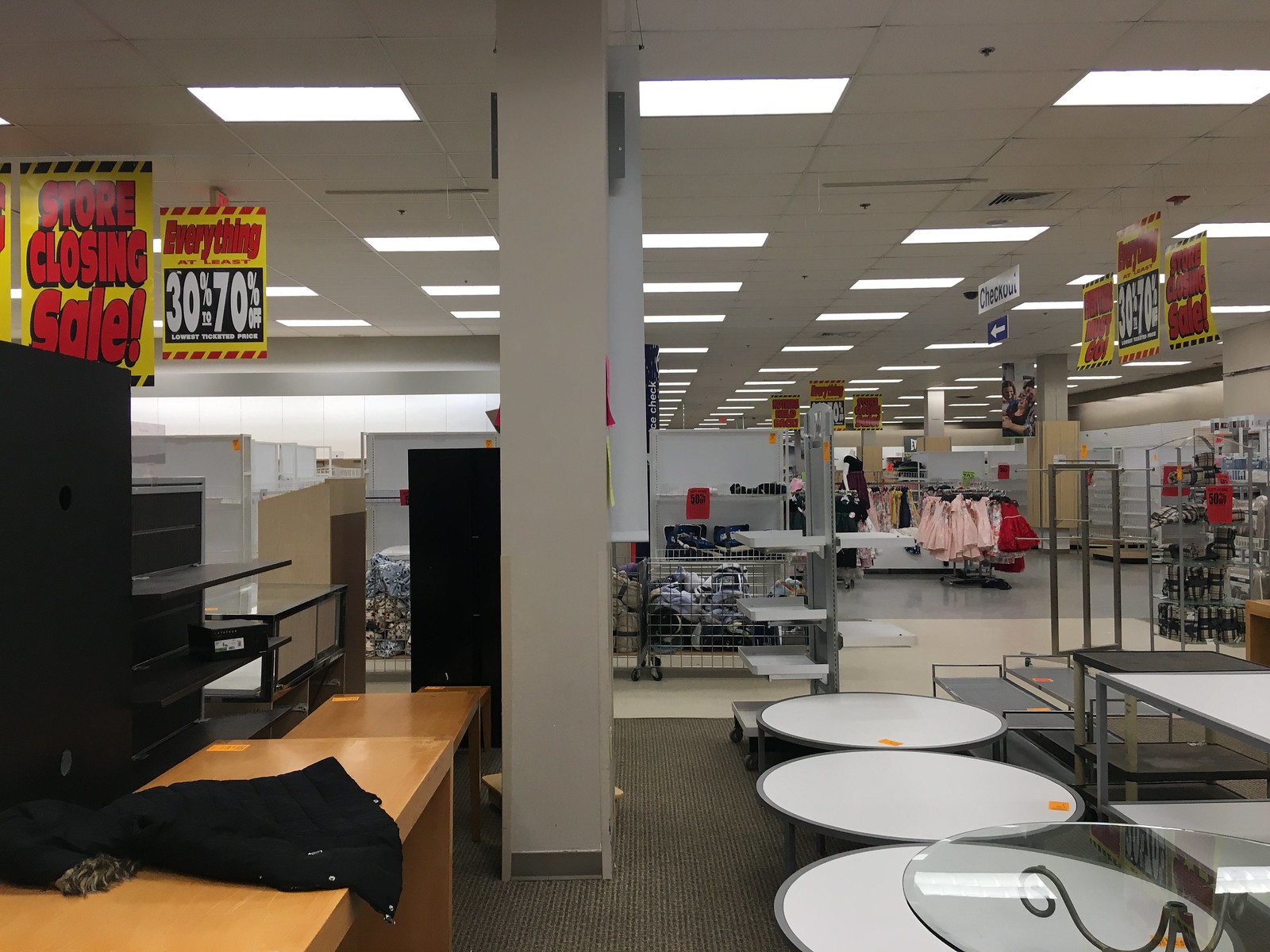This high-resolution color photograph captures the interior of a retail store undergoing a closeout sale. The ceiling is painted grey and fitted with square recessed lighting, and prominently features yellow signs with red and white text proclaiming "Store Closing Sale" with discounts ranging from 30 to 70%. Below these signs, black shelving units are visible, most of which are empty, indicating the extent of the sale. On the left side of the frame, a black object is draped over a wooden shelf, contributing to the sense of disarray typical of a store in its final days. A large, structural pillar descends from the ceiling, segmenting the space. To the right, three circular tables or bins, likely used for displaying discounted items, stand empty, each adorned with small tags that could be price markers. The lower right corner of the photograph shows the edge of a glass table. Central to the scene are bins filled with various items, while in the distant right, racks of hanging pink and red clothing are visible alongside shelves cluttered with small objects. Additional discount signs are suspended from the ceiling, further emphasizing the clearance event.